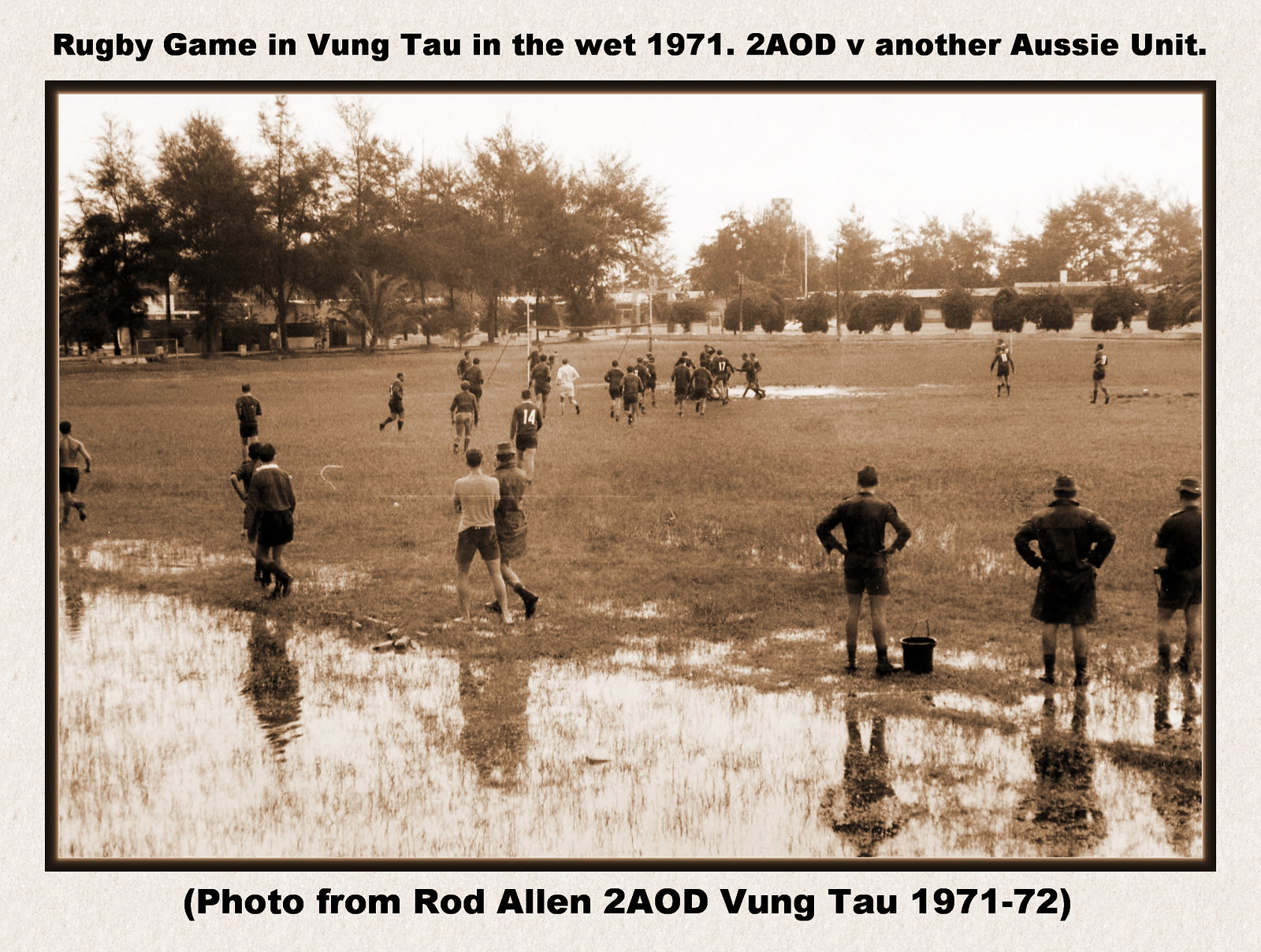The sepia-toned photograph captures a rugged rugby match taking place on a football field plagued with large puddles and muddy conditions, characteristic of Vung Tau in 1971. The players, roughly twenty in number, are dressed in dark uniforms with visible numbers on their backs, and they are densely clustered in the center of the image, a rugby ball barely discernible amidst the commotion. The poor state of the field is evident with waterlogged patches and visible grass struggling through the mire, forming a stark contrast to the backdrop of trees and bushes. Spectators, around seven or eight, are visibly standing along the sidelines, one notably with a bucket at his feet, observing the wet and chaotic game. The photograph is elegantly framed, featuring captions both at the top and bottom. The top reads, "Rugby game in Vung Tau in the wet, 1971, two AOD versus another Aussie unit," and the bottom text states, "Photo from Rod Allen, II AOD, Vung Tau, 1971-72."